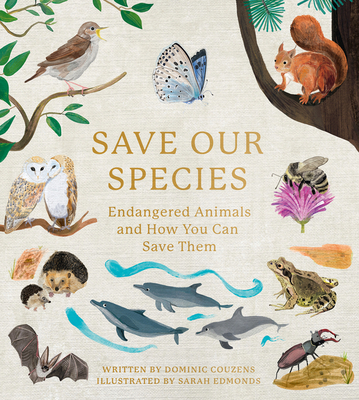The book cover of "Save Our Species: Endangered Animals and How You Can Save Them" is a captivating illustration against a cream-colored background. The title is prominently featured in yellow font in the center, flanked by various endangered animals intricately illustrated throughout the cover. In the upper left corner, a brown bird with a white body and a yellow beak perches on a leafy tree branch. Directly to the right is a vividly blue and white butterfly in flight. A brown squirrel is perched on a branch in the upper right corner, peeking through the leaves.

Below the title, on the left side, two owls are comfortably settled on a branch. Nearby, there are two hedgehogs, one appearing to be a mother with her baby, and what seems to be opossums or similar small rodents. To the right of the title, a bee is busy pollinating a pink flower, and under it, a green and black spotted frog is perched. Continuing right, a pink and gray beetle, possibly a Hercules beetle, is positioned in the lower right corner. 

At the bottom of the book cover, three dolphins are illustrated swimming in a group. Nearby, a bat with a white chest is seen flying in the lower left corner. The center lower part of the cover states the author and illustrator: "Written by Dominic Couzens, Illustrated by Sarah Edmonds," with precise detail ensuring Sarah is spelled with an H. Each element blends harmoniously to create a detailed and engaging image, emphasizing the beauty and diversity of endangered species featured in the book.